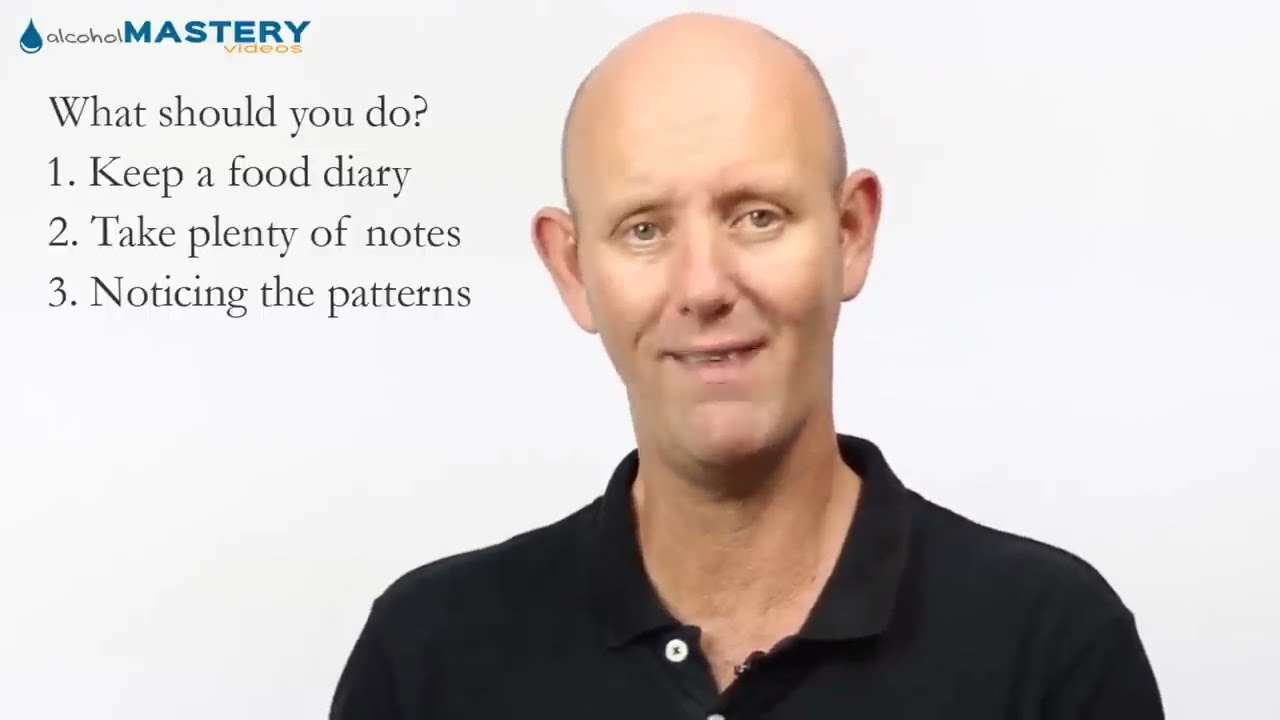This advertisement, likely a brochure for a self-help organization focused on overcoming alcohol addiction, features a prominent image of a bald Caucasian man with a long face and large ears, who appears somewhat sickly and possibly jaundiced. He has a somewhat weak, partial smile, revealing some of his teeth, and wears a black polo shirt with white buttons and a microphone clipped to the collar. In the top left corner on a white background, a blue water droplet contains the word "ALCOHOL" in black writing, and "MASTERY" in blue writing. Below this, in orange font, it says "VIDEOS." Beneath that, the black text asks, "WHAT SHOULD YOU DO?" followed by a list: 1. KEEP A FOOD DIARY, 2. TAKE PLENTY OF NOTES, 3. NOTICING THE PATTERNS. The man appears to be the focal point of the advertisement, potentially addressing viewers about overcoming alcohol dependency.